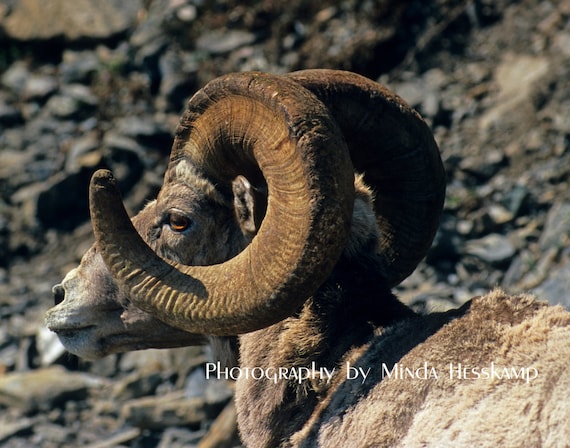This image captures a close-up side profile of a bighorn sheep, also referred to as a ram, set against a stark, rocky backdrop. Photographed by Minda Heskamp, the image is crisp and clear, emphasizing the detailed features of the sheep. The ram's large, curved horns cast a shadow on its body, circling almost all the way around to extend below and in front of its eye. The sheep is mostly brown, gray, and black, with an orangey-brown eye that looks to the viewer’s left. The background is blurred, highlighting the horned animal, which occupies a prominent, central position in the frame. Only part of the sheep’s body is visible, showcasing about half of it without any legs or hindquarters. The sun illuminates the animal, further dramatizing the rugged texture of its horns and the coarse details of its fur against the rocky setting.